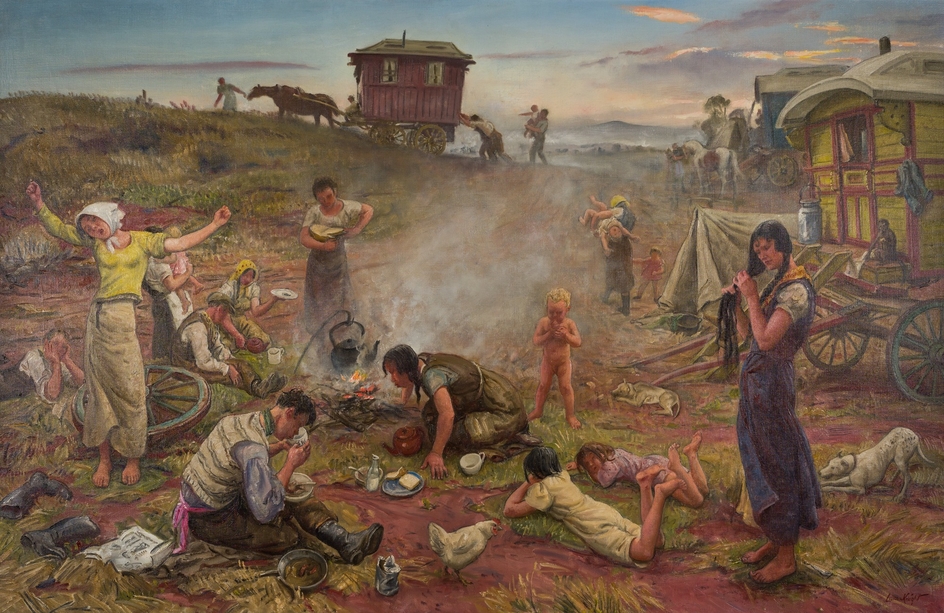The painting depicts a lively rural scene from the 1800s, illustrating settlers in the wilderness. In the foreground, a woman in a traditional blue dress with long black hair, who is braiding her hair, stands next to a lady in a yellow shirt and skirt with a white bonnet stretching her arms. Nearby, a man in a white vest, blue shirt, and brown pants sits cross-legged, eating and drinking. Children, including two girls lying on their stomachs with legs crossed and a young blonde boy standing naked, are scattered around, adding to the vibrancy of the scene. Centered around a campfire, where a woman in a plain brown dress tends a black kettle hanging over the fire, the settlers are engaged in their daily activities.

In the background, multiple trolleys or carriages with large wheels, some painted in bright colors like yellow, blue, and red, are either being pulled by horses or pushed by people across a reddish-yellow dirt road that cuts through patches of green grass. The settlers’ carriages serve as their mobile homes during their journey. The backdrop features a reddish-brown dirt expanse, a distant hill, and a bright blue sky with streaks of pale yellow, gray, and purplish-red clouds, all set against a setting sun. This impressionistic painting beautifully captures the essence and struggles of early settlers in the wilderness.